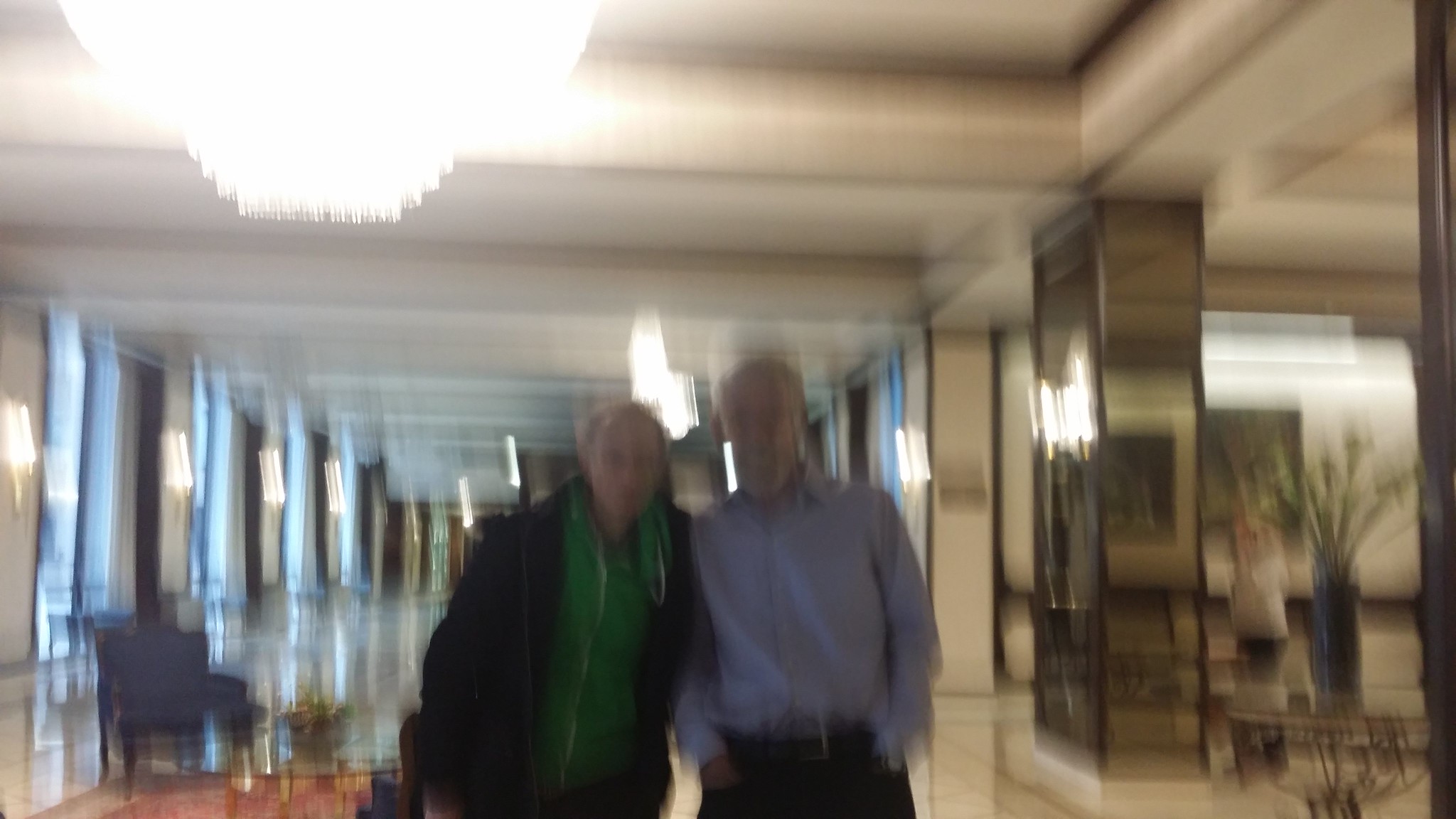This very blurry landscape photograph captures two men standing closely in what appears to be a vast and extravagant hotel lobby, filled with a sense of grandeur. The man on the left is bald, sporting a black coat over a green zip-up hoodie. Light reflects off his head as he leans in towards the man on the right, who has a gray beard and is also bald. The right-side figure is dressed in a bluish shirt with black pants, his hands casually tucked into his pockets, showcasing the silver outline of his belt buckle. The background reveals a luxurious setting with a giant chandelier shining brightly in the top-left corner, casting a white blur. Below it, a red rug features a blue chair with wooden legs. Mirrored columns, tall planters with lush plants, and an elegant stone floor add to the opulent ambiance, with large windows on the left side illuminating the space and leaving intricate reflections. In the distant back, a painting adorns the white wall, completing the sophisticated scene.